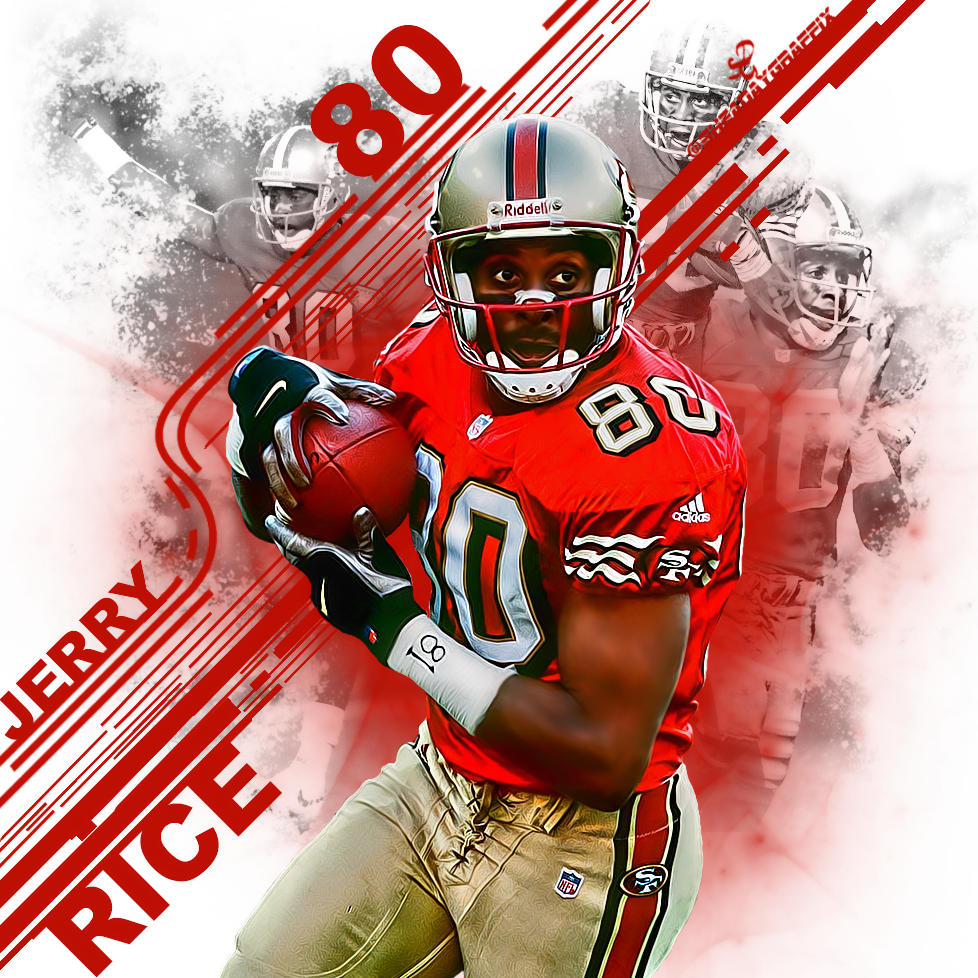The poster prominently features an American football player, identified as Jerry Rice, in the center. He is a black male, captured in mid-action, seemingly running while holding a red football. Jerry is dressed in a red sports jersey with the number 80 in white, paired with golden beige pants that have red and black stripes down the sides. His helmet is silver with a distinctive red stripe flanked by black stripes down the middle, adorned with the word "Riddell" in red. Notably, there is a white strip across his nose, and his gloves are black with silver accents, featuring the Nike logo.

The sleeve of his jersey shows the brand Adidas, and he also has a white armband with the number 81 visible on it. The background contains a black and white image of other players, adding depth to the composition. Red design lines adorn the image, along with prominent text to the left that reads "Jerry Rice 80" in matching red, affirming the player's legendary status.